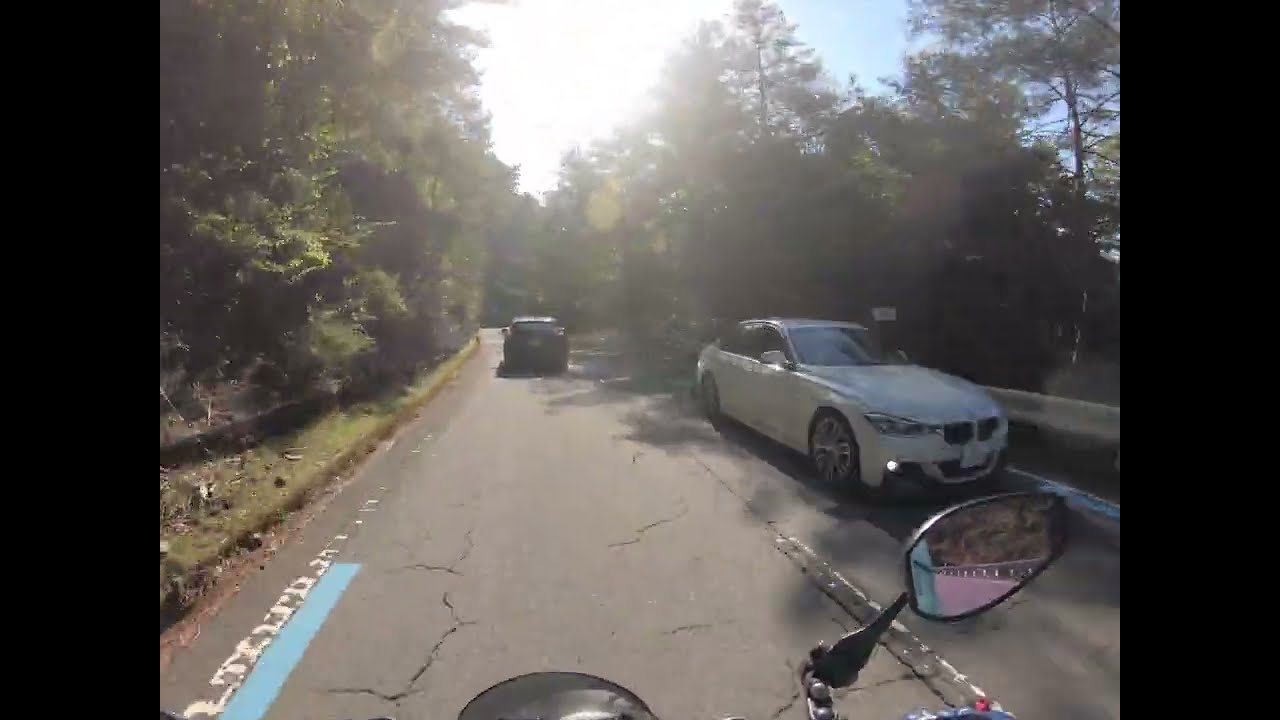This image captures a motorcyclist's point of view while riding on a two-lane road, likely taken with a GoPro camera. The road has one lane for each direction of traffic. Positioned at the bottom right is the motorcycle’s silver mirror, reflecting part of the road and surroundings. Ahead of the motorcyclist, in the same lane, is a black car. Coming towards the motorcyclist in the opposite lane is a white BMW sedan with five-spoked chrome metal rims. The photo suggests the rider might be in a country where traffic drives on the left side of the road, navigating a curvy, possibly mountainous terrain. Lush green trees flank both sides of the road, extending up to a clear blue sky, which features a bright sun situated in the top center of the image. The scene suggests an impending sharp left turn due to the curvy nature of the road. Despite some blur in the image, the vivid elements are clear, rendering a detailed and dynamic snapshot of the ride.